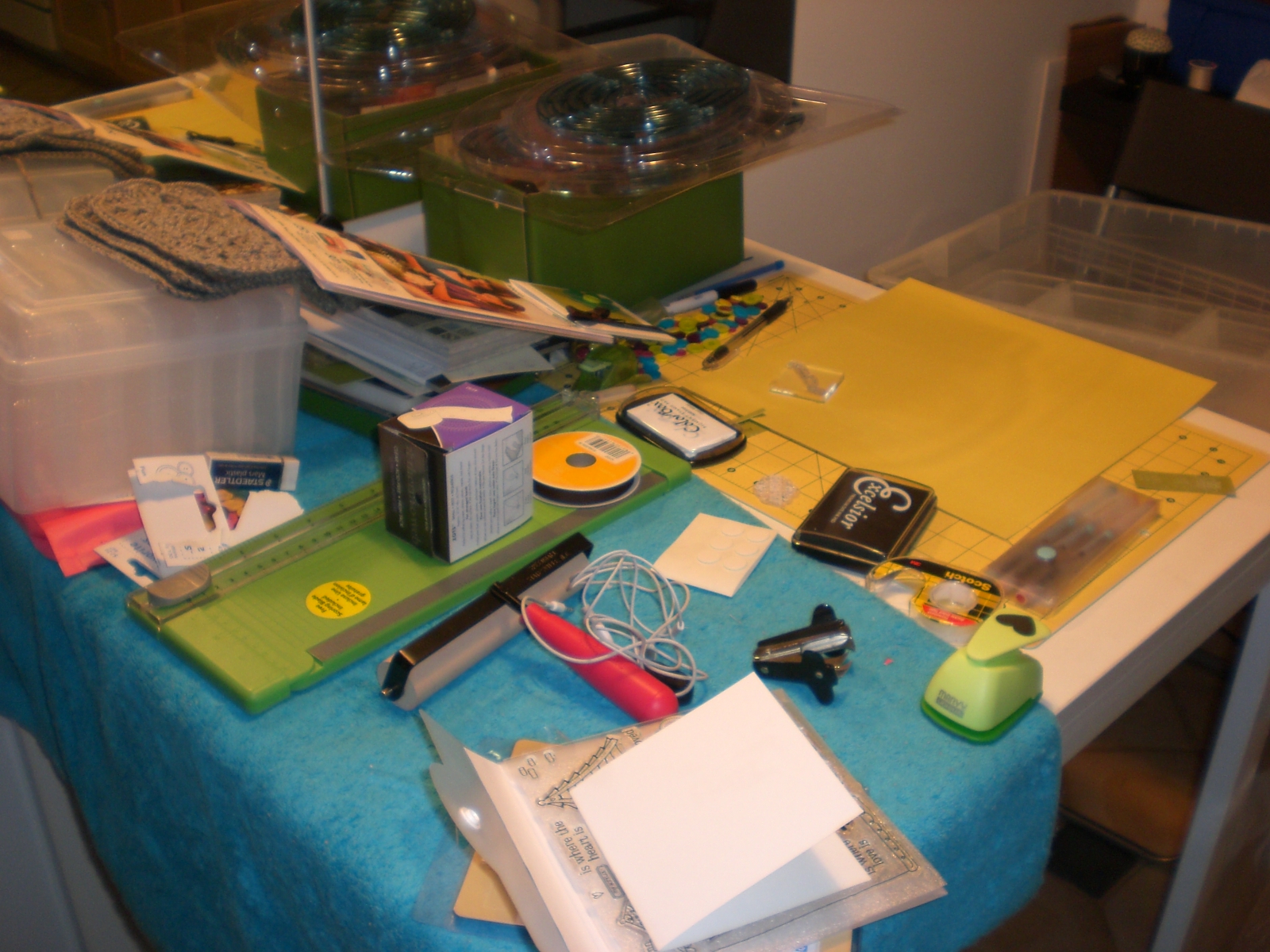In a dimly lit room with white walls, a cluttered table is laden with various items, suggesting it might be an arts and crafts workspace. The table is half-covered by a folded blue towel, while the other half reveals a white wooden surface. A plethora of stationery including pens, paper, tape, and a potential rubber stamp pad are scattered across the table. A squeegee or roller is also present amidst the clutter. On the towel-covered section, multiple boxes and a spool of ribbon are visible, alongside several Rubbermaid containers precariously stacked with magazines slipping off them. A green box topped with plastic packaging stands at the top center of the image. In the top right corner, items are haphazardly piled on top of each other. Additionally, a mirror reflecting some table contents adds to the disarray captured in this scene.